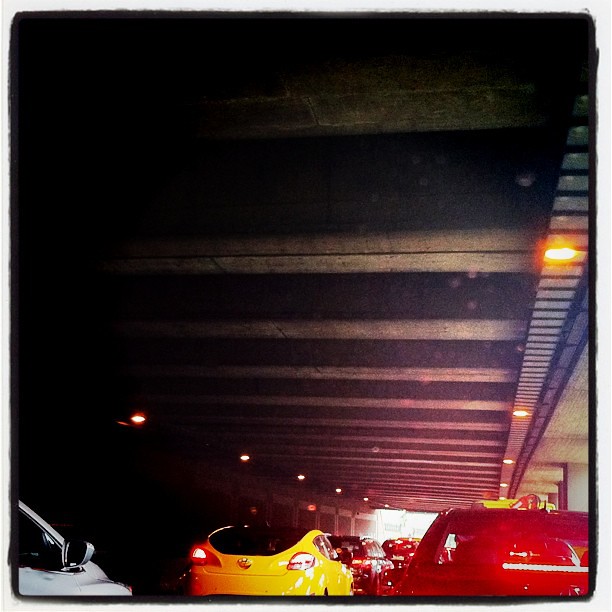The image depicts a congested traffic jam under a steel-beamed overpass or tunnel. The ceiling is black with long gray beams and is equipped with periodically spaced, bright orange, rectangular lights set into it. Tail lights from the numerous vehicles create a sea of red, indicating that the cars are braking. Notable vehicles include a yellow sports car in the center with one tail light out, a white car further ahead almost at the end of the tunnel, and another car on the right with a long rectangular back window. Off in the distance, daylight is visible, suggesting the tunnel is ending, although traffic likely continues beyond it. The entire scene is vividly lit by the car headlights reflecting off one another, and the blurred rear view of vehicles further highlights the congestion.